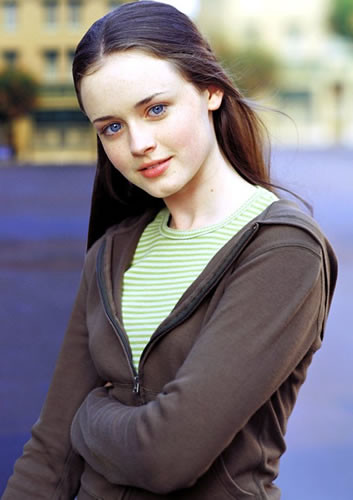In this promotional photo, a young woman, possibly an actress, is captured posing in the center. She has long, neatly parted brown hair that reaches below her shoulder blades and striking blue eyes. She slightly smiles at the camera, adding a touch of warmth to her expression. Dressed in a green and white striped crewneck shirt with very slim stripes, she wears a dark gray zip-up hoodie over it. Her casual yet thoughtful pose includes her left arm folded across her midsection while her right arm hangs naturally at her side. 

The background is blurred but suggests an outdoor scene with tall buildings that have numerous windows and are at least two to three stories high. Adding to the urban landscape, trees are visible on both sides of the buildings. There seems to be a patch of blue, likely representing water, and a brownish area that could either be a road or a paved area. The overall setting suggests an urban environment with a mix of natural and man-made elements, enhancing the sense of depth in the photo.